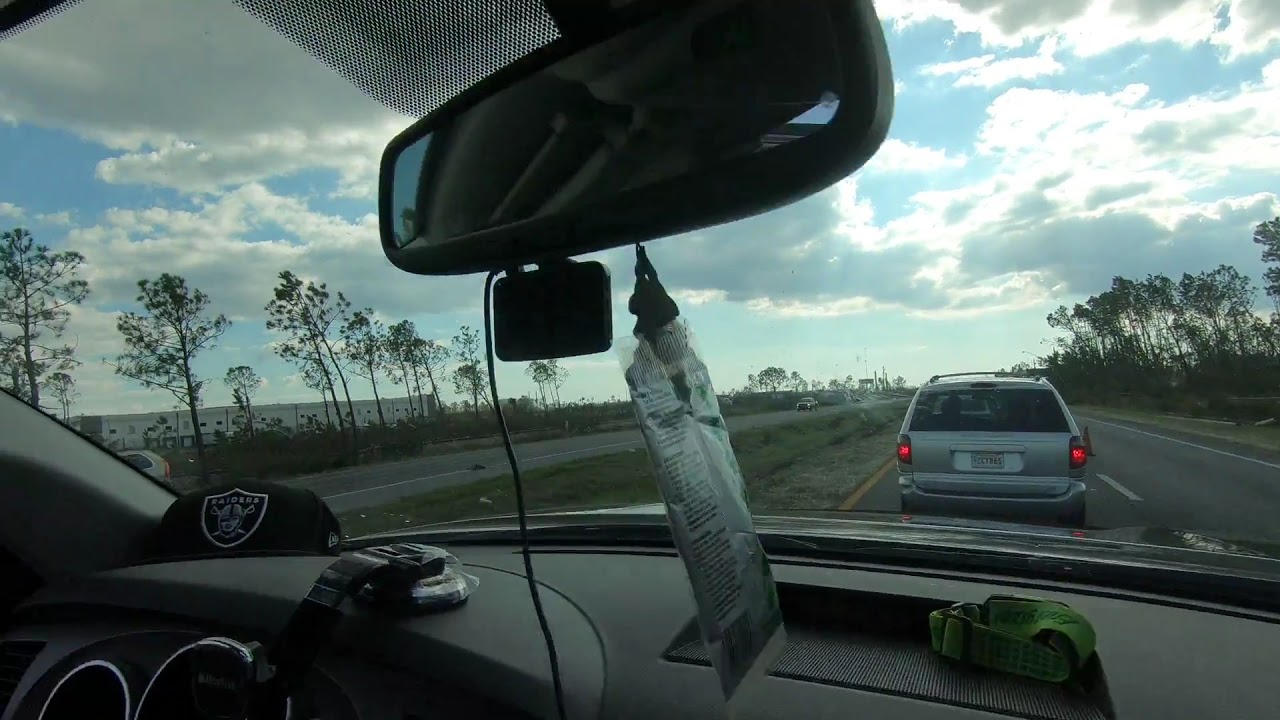The image captures a scene from within a car, presumably taken from the passenger side but possibly from the driver's perspective, extending their arm to the right. In front of this car is another vehicle—possibly a van, minivan, or small SUV—driving closely ahead. The brake lights of this silver vehicle in front are illuminated. The road stretches forward in a northbound direction, with an opposite lane to the left, alongside some greenery and lined with trees. To the left of the road are buildings that appear to be either apartments or offices.

The sky is predominantly blue with numerous white clouds. Inside the car, several details are visible: the dashboard holds a black Raiders hat, and from the rearview mirror hangs an air freshener. There is also a lanyard or strap visible on the dashboard. The bright daylight setting and clear weather conditions contribute to the overall brightness and clarity of the image. There are no people visible in the scene, emphasizing the peaceful, almost still-life quality of the photograph.